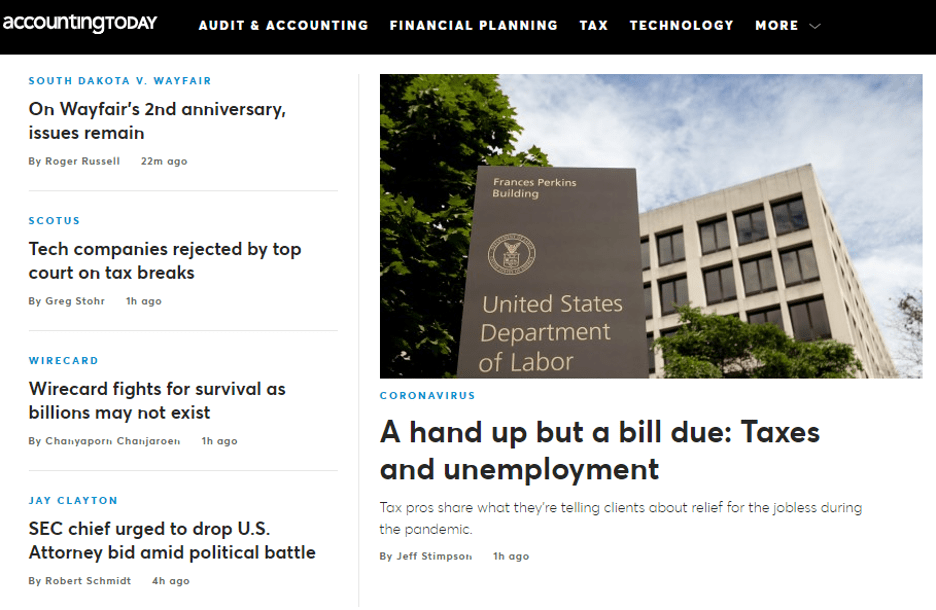The "Accounting Today" homepage features a sleek black navigation bar at the top with categories including Audit and Accounting, Financial Planning, Tax, Technology, and more. On the left side, the page displays a selection of articles, with the central focus on a main article prominently featured towards the bottom right. This main article, titled "A Hand Up, But a Bill Due: Taxes and Unemployment," discusses tax advice provided to clients regarding relief for the unemployed during the pandemic. The article is accompanied by an image of the exterior of the somber Francis Perkins Building, a part of the Department of Labor, possibly its headquarters.

To the left of the main article are additional headlines without images, including:

- "On Wavier's Second Anniversary, Issues Remain"
- "The Company is Rejected by Top Court on Tax Breaks"
- "Wirecard Fights for Survival as Billions May Not Exist"
- "SEC Chief Urged to Drop U.S. Attorney Bid Mid-Political Battle."

The page design features a clean, white background with black text, and articles are sometimes identified with tags or labels, such as a "coronavirus" tag on the main article.